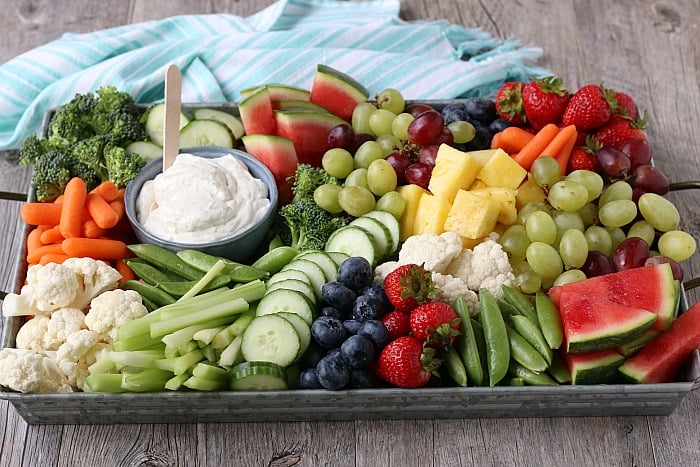The image depicts a professionally photographed, horizontally-aligned rectangular gray iron tray brimming with a vibrant and meticulously arranged assortment of fruits and vegetables. The tray is set atop aged, brown wooden planks, which could be either a floor or a table, adding a rustic charm to the scene. The background features a white and blue striped blanket or sheet, suggesting a cozy picnic setting.

Starting from the upper left corner of the tray, there is a lush bunch of broccoli, followed by a cascade of orange carrots and creamy white cauliflower in the lower left. A row of crisp, sliced cucumbers is adjacent, with a blue bowl of dip featuring a white stick nestled beside them. Fresh green snap peas and celery sticks add to the array of greens.

In the middle section, the top showcases succulent slices of watermelon, clusters of green grapes, another spread of broccoli, and more cucumber slices. Moving along, there are vivid red grapes, golden pineapple chunks, additional cauliflower florets, juicy strawberries, and tiny, plump blueberries.

The upper right of the tray continues the colorful feast with more strawberries and carrots, mingled with red and green grapes. The lower right corner is anchored by another round of refreshing watermelon slices. The scene includes a myriad of colors such as black, white, gray, blue, green, orange, off-white, yellow, purple, and red, making the platter as visually appealing as it is nutritious.